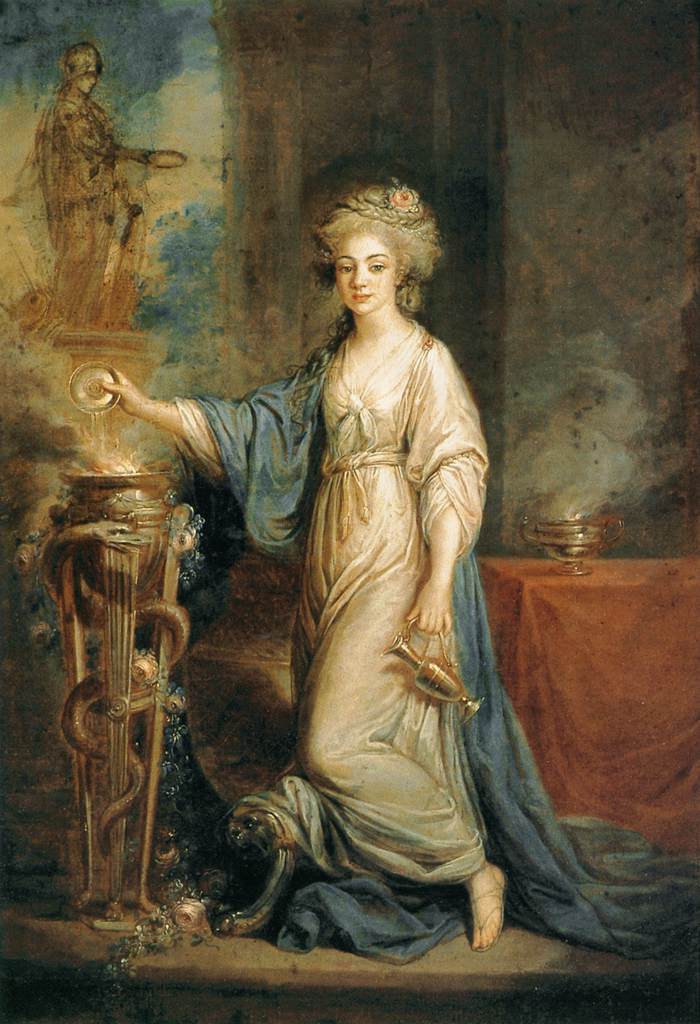The painting depicts a Renaissance-era European woman with long, flowing blonde hair neatly adorned with a flower. She is elegantly attired in a flowing white satin dress and a blue robe draped over one shoulder, trailing behind her. The woman stands poised, her body angled slightly to the left, with her bent knee and sandal-clad foot subtly highlighting her graceful stance. In her right hand, she holds a gold decanter by her side, while her left hand pours liquid from a cup onto a flaming pedestal, possibly a censer with a snake motif winding up its legs. The background features a red tablecloth-covered table, a genie lamp, and a painting that appears to depict a military scene or figure, completing the rich and intricate setting.